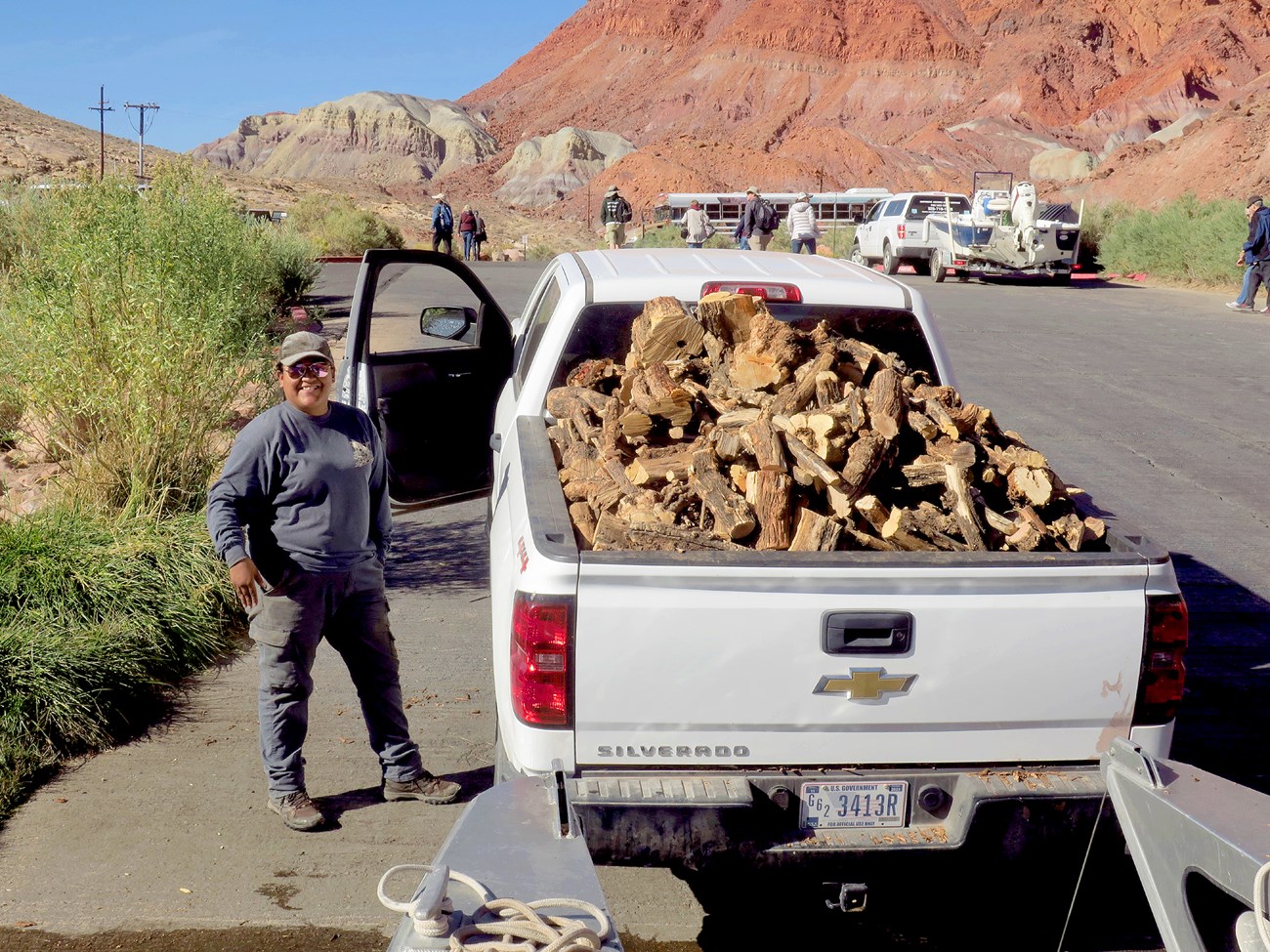In a deserty, clay mountain landscape, a bustling parking area is captured in the photograph. The main focus is on a large white Chevy Silverado truck, positioned on the side of the road, with its driver's side door open. The truck bed is stacked high with cut wood, possibly firewood or dead trees being cleaned up. Standing next to the truck is a person, possibly Hispanic, dressed in work clothes: jeans, work shoes, a long-sleeve t-shirt, a cap, and aviator sunglasses, smiling at the camera. In the background, nine people are scattered around, some near their vehicles, including a large grey school bus and another truck pulling a boat trailer. The scene is framed by deserty reddish clay mountains and green shrubs under a bright blue sky. The Silverado sports a U.S. government license plate, indicating an official capacity for the gathering.